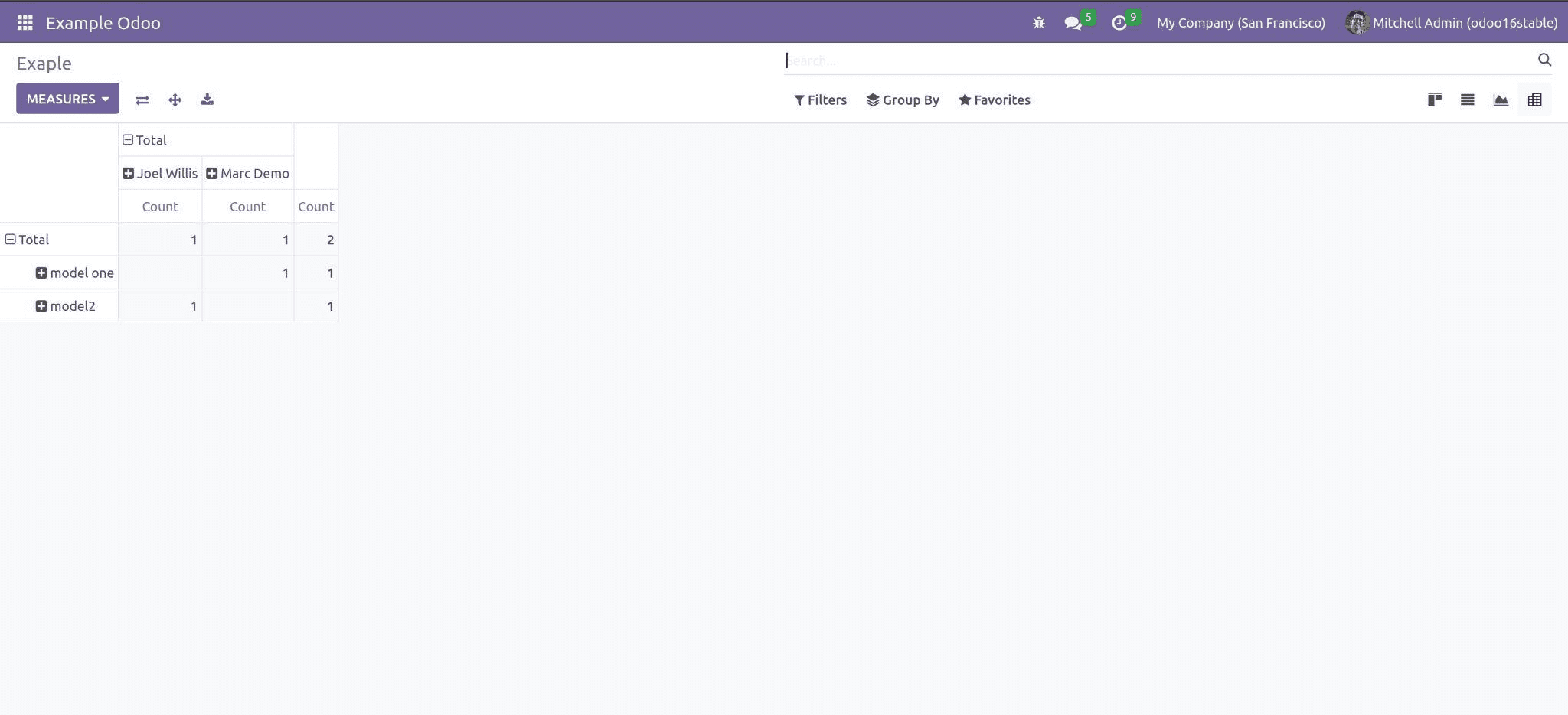The website interface displays "Example Odoo" prominently on the top left, with "Odoo" spelled O-D-O-O. Adjacent to this label, on the right, is a messaging icon indicating 5 unread messages in green. Next to the messaging icon is a clock symbol showing the number 9 in green. Further to the right, the text reads "My Company (San Francisco)," indicating the company and location. The profile section features the user name "Mitchell Admin," followed by "odoo 16 stable" in parentheses, denoting the software version.

Central to the display is a spreadsheet-style interface reminiscent of Excel, featuring various columns and rows for detailed data analysis. Rows are labeled "Model 1" and "Model 2," while columns are labeled "Joel Wills" and "Mark Demo." There is also a "Count" column listing numbers ranging from 1 to 2. Totals are calculated and displayed on both the right-hand side of the columns and the bottom of the rows.

Above the spreadsheet, a prominent purple "Measures" button is available. The interface includes sections for filters, group-by options, and favorites, enabling customization of the data view. There's also a search bar with a magnifying glass icon for quick, specific queries.

The background color of the webpage is a subtle grayish-white, providing a neutral backdrop, while the toolbar at the top stands out in purple, adding a vibrant touch to the otherwise muted aesthetic.